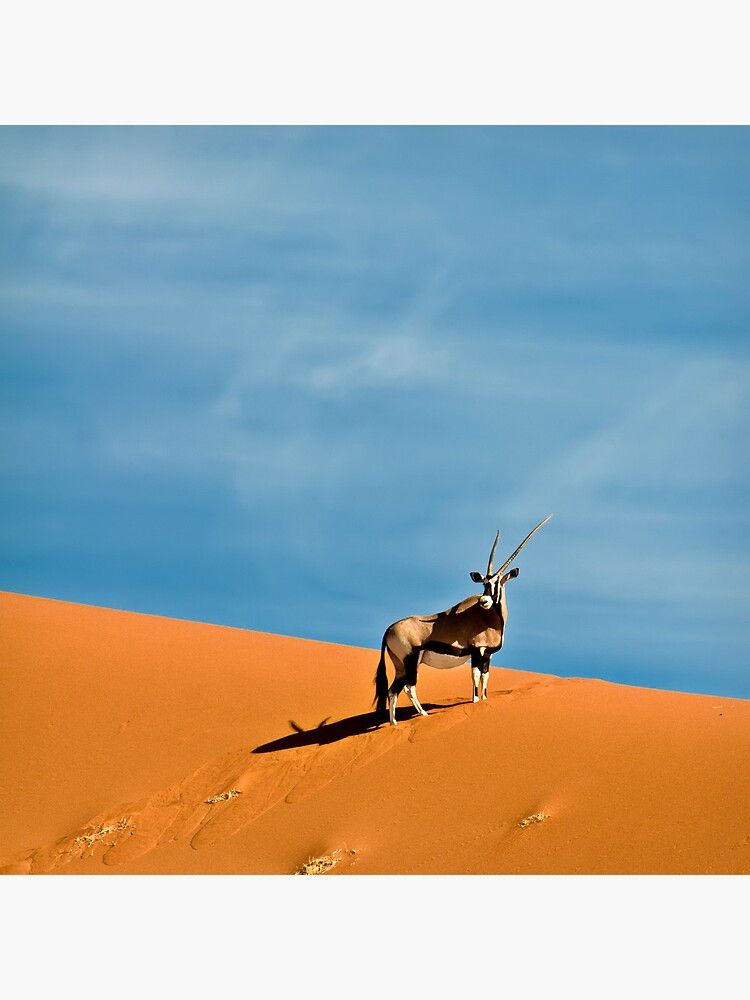This is a detailed photograph of an ibex standing majestically on a dark reddish-orange sand dune, likely in a desert. The ibex is positioned in the bottom quadrant of the image, with its striking silhouette against a vast, bright blue sky that occupies about two-thirds of the frame. Wispy, faint white clouds streak the sky, adding to the desolate yet captivating scenery. The ibex, with its long, tan, V-shaped horns, appears to be gazing over its right shoulder towards the bottom left corner of the photo. The animal's coat features a fascinating array of colors: a dark brown back, a white snout with black markings, a white stomach separated from the brown fur by a distinctive black line, white legs, and a black chest. Its long tail ends in a fluffy tuft, further accentuating its regal presence. Standing on the sienna-colored sand dune, the ibex exudes a sense of strength and grace amidst its barren surroundings.